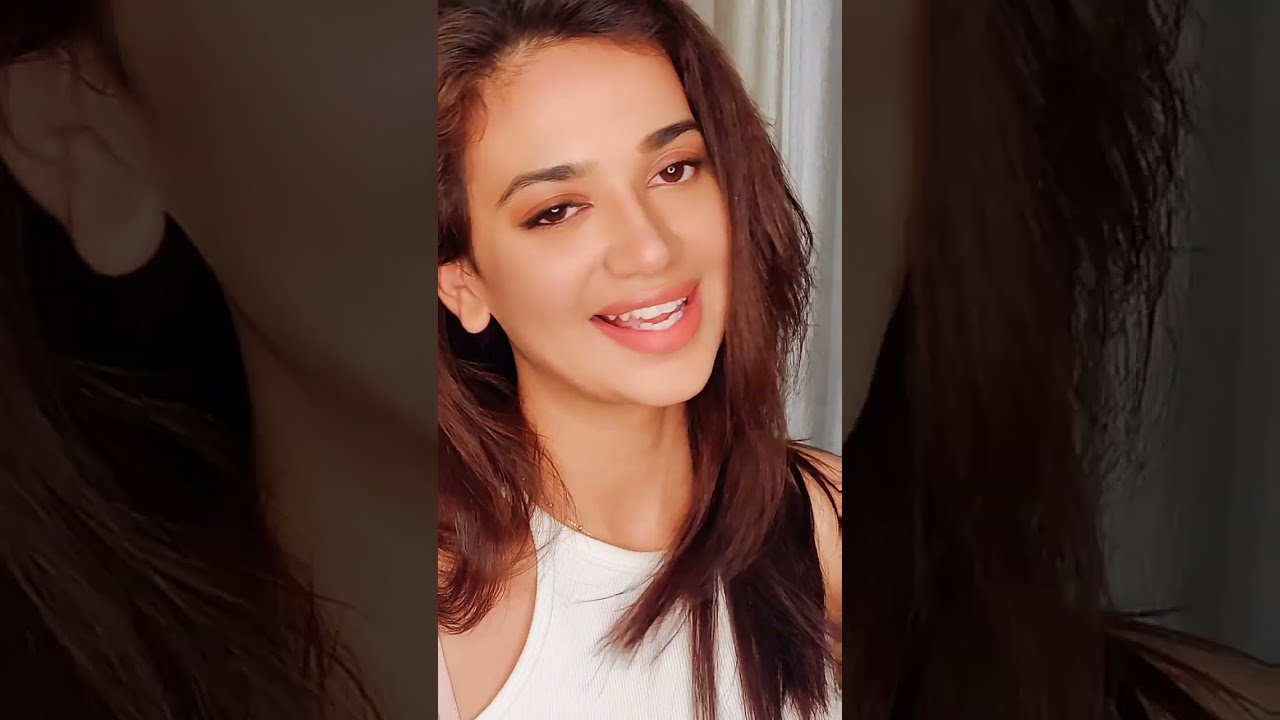This image is a close-up photograph of a woman taken indoors, likely during the daytime in a well-lit room. The woman takes up the entirety of the image and is positioned centrally. She has an olive skin tone and dark brown hair with subtle red highlights, which is pushed back from her forehead and tucked behind her ear on the right side. Her hair frames her face with wisps falling around her forehead and layers cascading over her shoulders and chest. 

The woman is wearing a white racerback tank top, and a hint of a gold chain necklace is visible, peeking from under the top. Her head is tilted slightly to the left, and she is looking directly at the camera with a smile that reveals both rows of teeth and a bit of her tongue, suggesting she might be speaking. Her makeup is neatly applied, enhancing her features. 

In the background, you can see a doorway with white trim. The image appears to be taken from a mobile device, resembling a screenshot from a social media app like TikTok or Instagram.